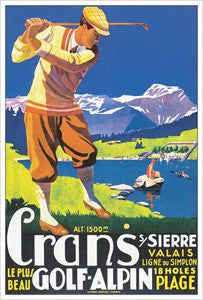This vintage-looking poster depicts a golfer mid-swing, dressed in a classic attire featuring a checkered yellow cap, a beige golf sweater with horizontal orange and white stripes at the bottom, baggy brown pantaloons, white stockings, and brown shoes. The golfer stands against a scenic backdrop, which includes a river on the right, a plot of grass above it, a line of trees on the horizon, and majestic, snowy mountains under a clear blue sky. Additionally, a woman can be seen sitting on a rock towards the center-right of the image. At the bottom of the poster, there's prominent white text reading "Kranz / Sierre," followed by yellow text "Valais." Below that, it says "Ligny du Simplon," and to the bottom right, "Les Plus Beaux / BAU." There's also a bullet point symbol, beside which in yellow text it says "18 holes." The word "Plage" is noted at the very bottom.